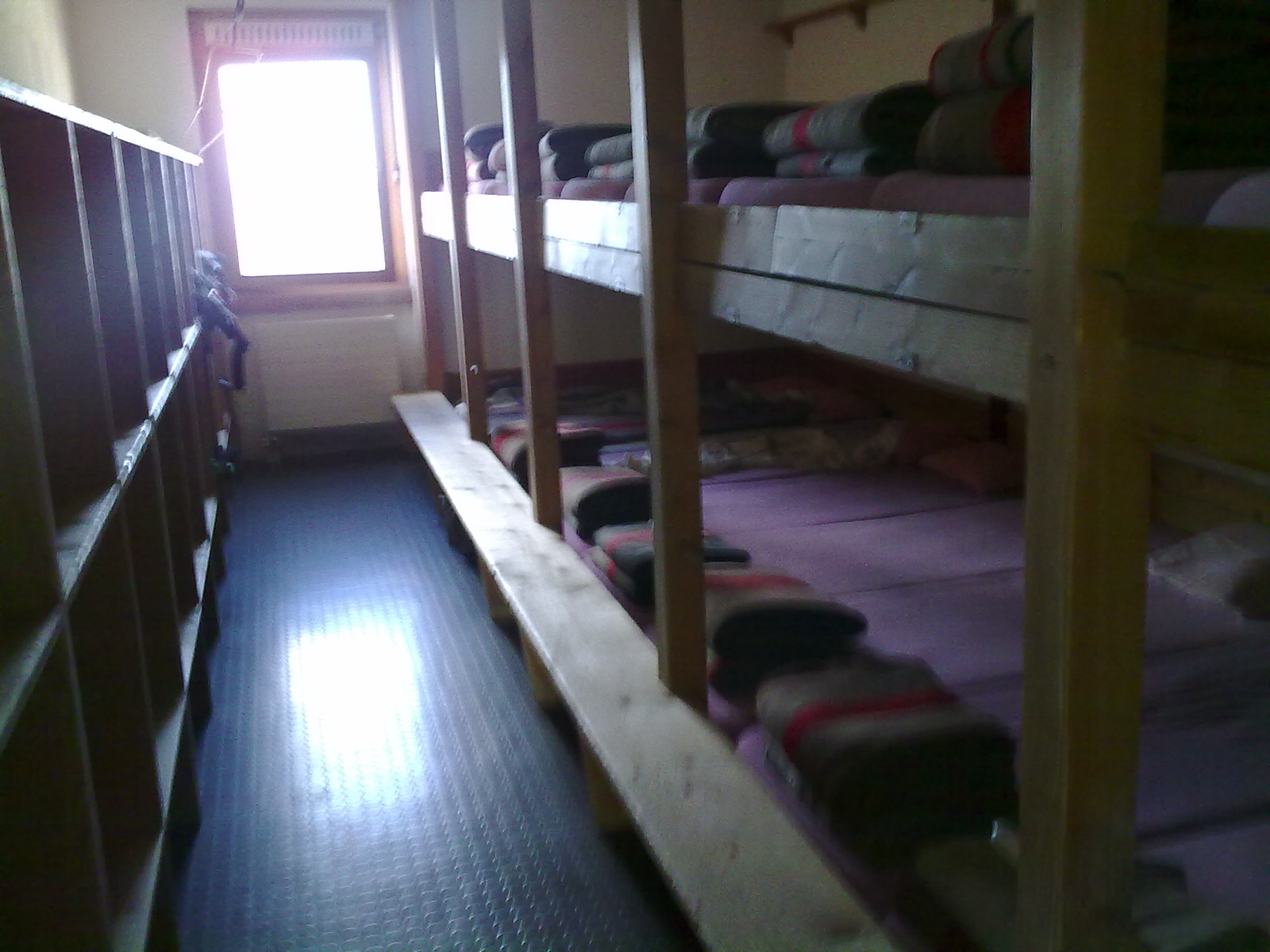The photograph captures a room adorned with dormitory-style sleeping arrangements. On the right-hand side, a long set of wooden bunk beds spans the length of the wall, crafted from light wood and arranged in two stories. Each bed is neatly outfitted with a lavender mattress, upon which rest pink blankets, with additional folded beige blankets featuring a red stripe placed at the foot of each bed. This configuration is mirrored on both the top and bottom rows. Opposite the bunk beds, the left wall is lined with a grid of wooden cubbies, providing storage space. The room is sectioned by a small walkway between the bunks and cubbies. At the back, a rectangular window allows sunlight to stream in, illuminating the tile floor and casting a bright beam of light down the walkway. Despite the image's blurriness, one can discern pillows on some beds and a white object situated above the window, where the sunlight emanates from. The overall ambiance suggests a functional, albeit spartan, sleeping area.